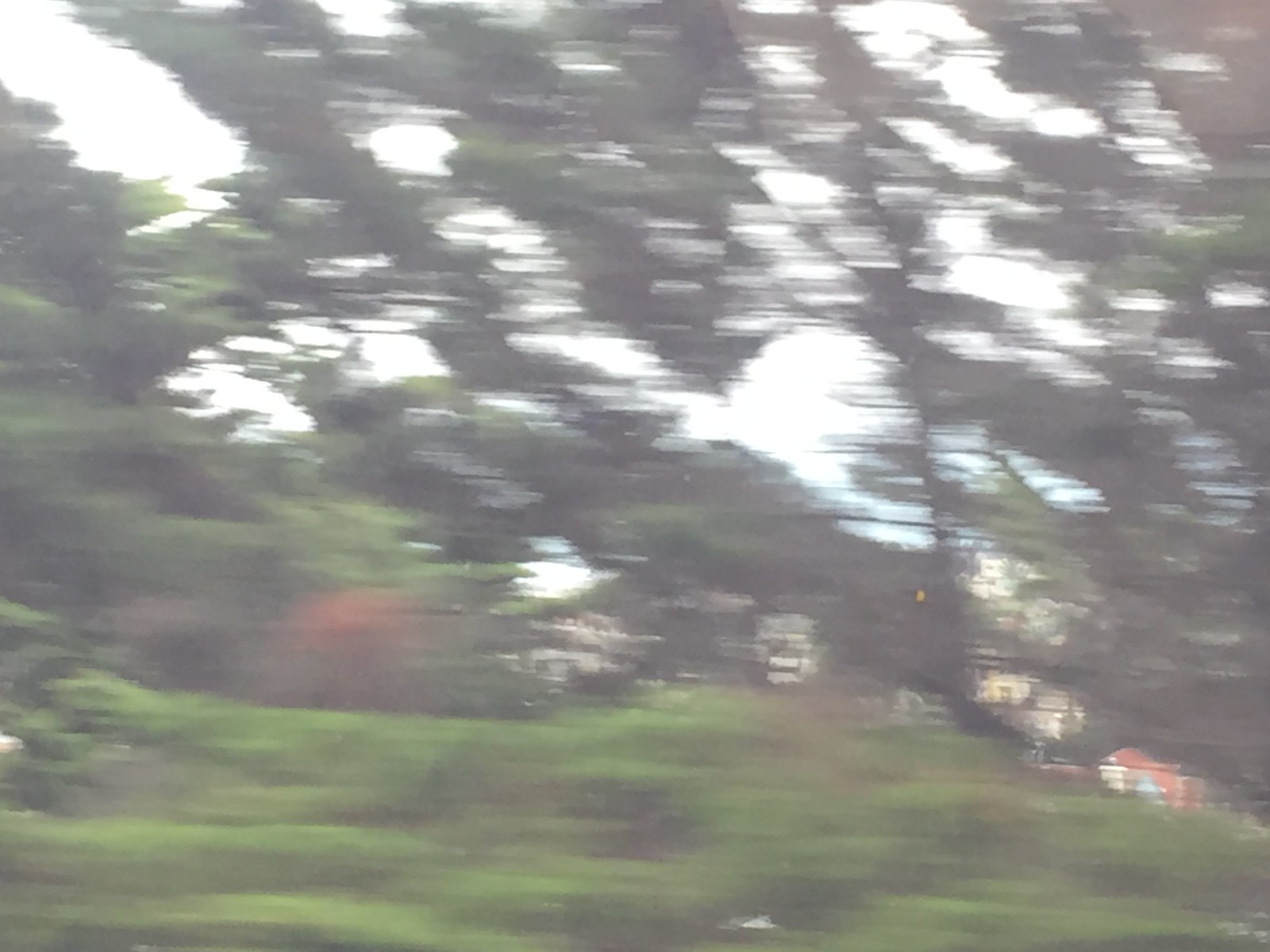A blurred image, likely captured from a moving vehicle during daytime, showcases a dynamic landscape of tall evergreen trees in shades of dark green and black, with the camera panning from left to right. The lower section is dotted with lighter, brighter green shrubs and bushes, interspersed with hints of orange and brown. In the distance, partially obscured by the trees, stand a few buildings in contrasting hues of yellow, white, and orange. Above, the sky is predominantly overcast with a blanket of white clouds, though a small patch of blue sky peeks through near the bottom middle right.